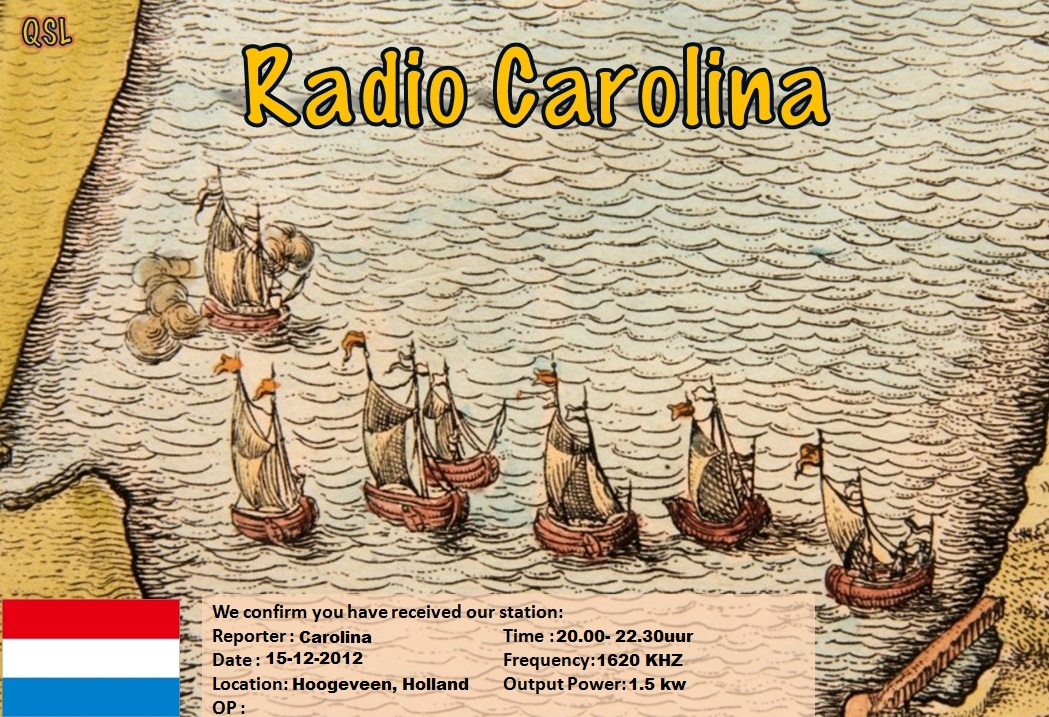The image is a colorful, cartoony illustration depicting seven sailboats traversing a wavy blue ocean, flanked by brown shorelines on both sides, reminiscent of an old-timey map. The scene is framed by significant textual details that enhance its narrative. In the top-left corner, the initials "QSL" appear in a playful, almost comic sans-like font, while the center-top prominently features the title "Radio Carolina" in yellow letters. At the bottom-left corner, a red, white, and blue flag—likely of Spain—is displayed beside a text box containing confirmation of reception details: "We confirm you have received our station. Reporter Carolina, date 15-12-2012, location Hoogeveen, Holland, time 20:22, frequency 1620 kHz, output power 1.5 kW." The entire composition conveys a whimsical yet informative atmosphere, combining maritime imagery with broadcasting elements.